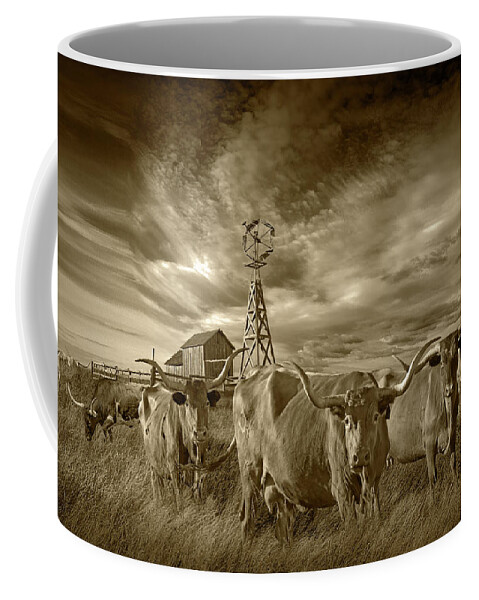This is a detailed close-up photo of a white mug with a sepia-toned design printed on it. The design prominently features a group of longhorn cattle—four or five in total—grazing on a grassy pasture. These cattle, with their distinctive two horns, appear to be staring directly into the camera. In the background, there's a wooden barn with a fence around it, encapsulating a typical farm setting. Additionally, there's a tall structure nearby, possibly a cell tower or weather vane. The sky above is dramatic, filled with streaky, intense clouds that give a sense of turbulent weather. The overall design is rendered in a dark yellowish, gloomy tone, enhancing the rustic atmosphere of the pastoral scene depicted on the mug.